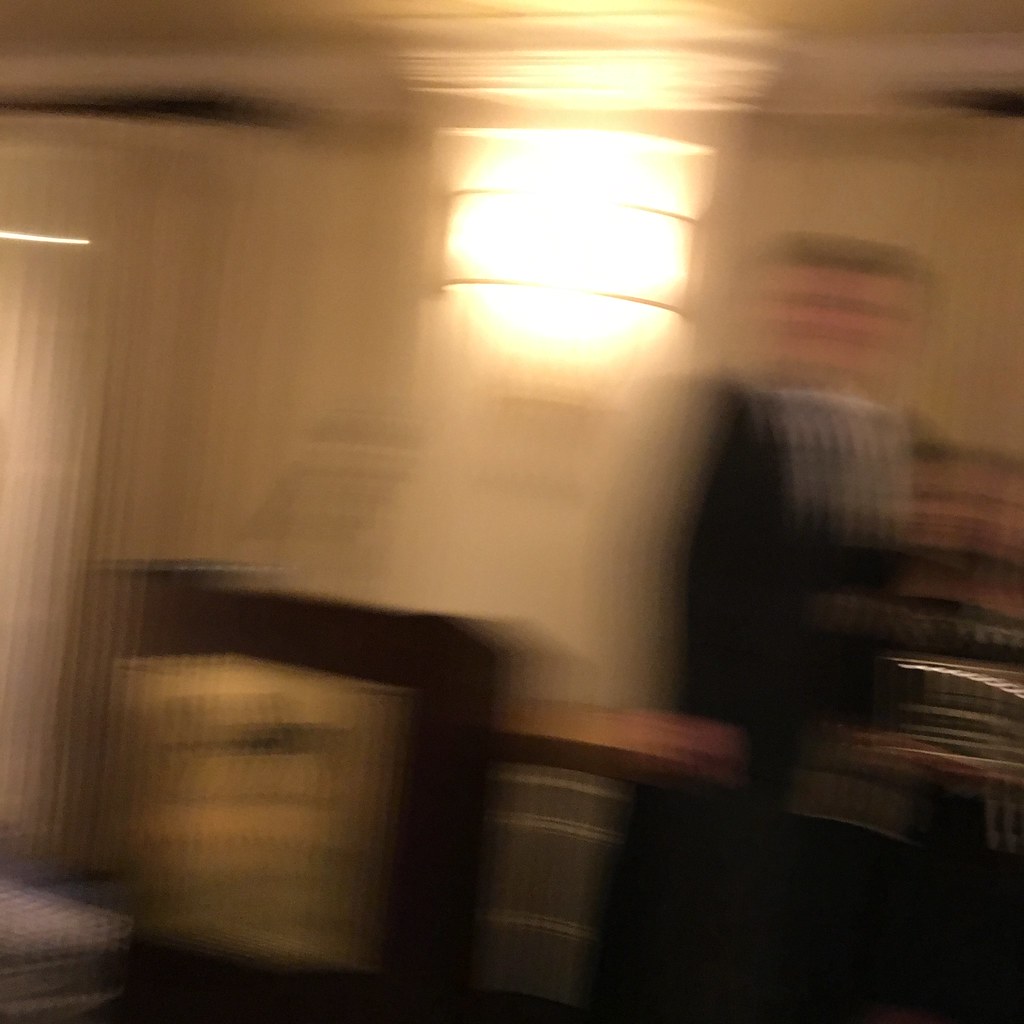A highly blurry digital photograph predominantly showcases an indistinct cream-colored ceiling in the upper left corner, transitioning into a cream-colored wall. A white running board can be seen extending horizontally from left to right. Near the top center of the image, an intensely bright area suggests yellowish sunlight streaming through a window, creating a vivid reflection. The left side of the photo is largely obscured by dark blurs, with something white partially visible just to the right of the bottom left corner. Adjacent to this, a black square is noticeable, adorned with a smaller yellow or gold square within it. There is also a red square next to these colored elements. To the right-hand side of the image, the visual information becomes increasingly ambiguous, filled with indistinct shapes and a mix of black, blue, and gray hues. The exact nature of these shapes remains unclear.